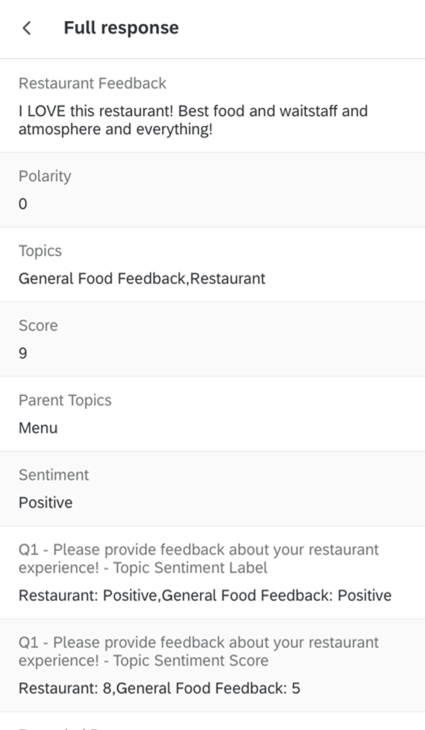**Caption:**

A pristine, white-background image showcasing a restaurant survey response. The feedback, filled with enthusiasm and love for the establishment, highlights the exceptional food, attentive wait staff, and delightful atmosphere. An exclamation mark underscores the diners' passion: "I love, love this restaurant!" The sentiment is clearly positive, with detailed praise for general food quality and overall restaurant experience. The survey questions are aimed at gathering comprehensive feedback, emphasizing positive sentiment and satisfaction. The image also displays scores, with the restaurant receiving an '8' for overall experience and a '5' for general food feedback.